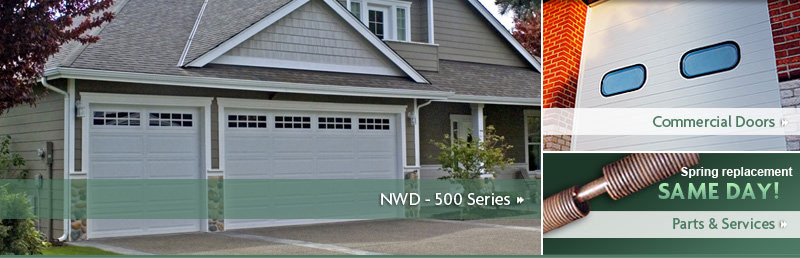The image is laid out in a landscape orientation and is divided into a larger section on the left and two smaller sections on the right. 

The left side of the image, which takes up two-thirds of the space, features a photograph of the front facade of a grey American-style house. This house has a double garage with a white door adorned with small windows at the top. Adjacent to this is a single garage door that matches the design of the double garage. The house’s exterior is painted in various shades of grey, reminiscent of a house from the video game "The Sims." Overlaying this photo is a semi-transparent green strip with the text "NWD-500 Series" written in white, accompanied by a small double arrow pointing to the right.

On the right side, the remaining one-third of the image is split into two unequal sections. The top section, which is larger, shows a close-up view of a commercial door. The door is white with two almost rectangular light blue windows that have rounded edges and black outlines. Over the image is the text "Commercial Doors." Below this, the smaller bottom section contains the text "Spring Replacement - Same Day! Parts and services."